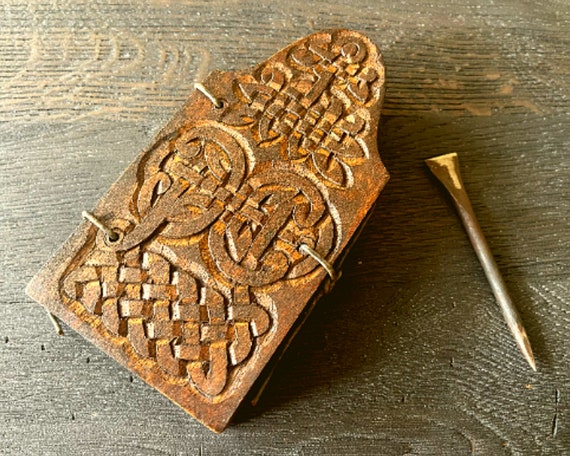The image shows a close-up of an ornate, rectangular metal plate with a slightly arched top, positioned on a brown wooden surface. The object features intricate carvings and a blend of decorative elements. The plate appears to be made from a rust-colored metal, possibly copper or an aged alloy, accented with yellow and dark brown touches. It is pierced with three holes—two on one side and one in the middle on the other, suggesting it might have been used for mounting or securing purposes.

The metal plate showcases a complex design with a woven pattern at both the bottom and top sections. In the middle, there are two ornate, backward C-shaped carvings facing each other. The top portion of the plate curves into a rounded point, embellished with patterns that resemble either a knot or a floral motif.

Resting next to this antique-looking plate is a large metal nail, characterized by a flat, yellow-tinted head, likely from hammering, and a pointed tip. The nail may have been used as a carving tool given its detailed description, adding to the sense of historical craftsmanship captured in this image.